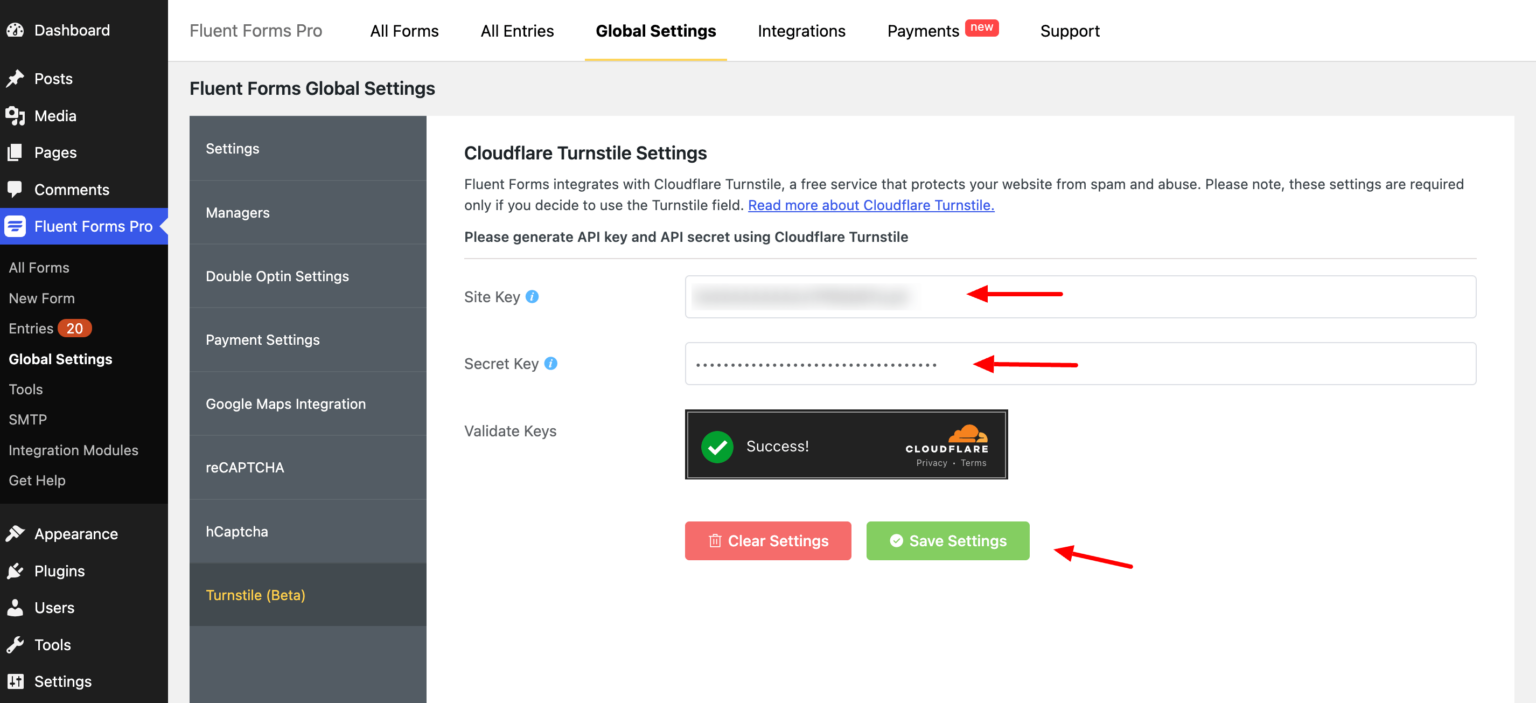**Detailed Caption:**

This image features a detailed screenshot of the Fluent Forms global settings interface. The webpage displays various configuration options pertinent to managing forms and security settings on a website. The section prominently highlighted in the interface is "Cloudflare Turnstile Settings," indicating that Fluent Forms integrates with Cloudflare Turnstile, a free service aimed at protecting the site from spam and abuse.

In the Cloudflare Turnstile settings, users are prompted with instructions to generate an API key and an API secret through Cloudflare Turnstile. The form includes fields for entering the site key and the secret key; however, the site key is grayed out while the secret key is concealed with dots, ensuring privacy. Options to validate, clear, or save these settings are provided.

To the left of the page, a vertical menu lists different navigational options available through the Fluent Forms Pro software. These include: Dashboard, Posts, Media, Pages, Comments, Fluent Forms Pro (further subdivided into All Forms, New Form, and Entries, with an example showing 20 entries), Global Settings, Tools, SMTP, Integration Modules, Get Help, Appearance, Plugins, Users, and Settings. 

At the top of the page, there is an additional horizontal menu specific to Fluent Forms Pro displaying categories such as All Forms, All Entries, Global Settings, Integrations, Payments, and Support. 

The interface aims to provide a comprehensive control panel for users to manage their forms and integrate necessary security features to enhance website protection.